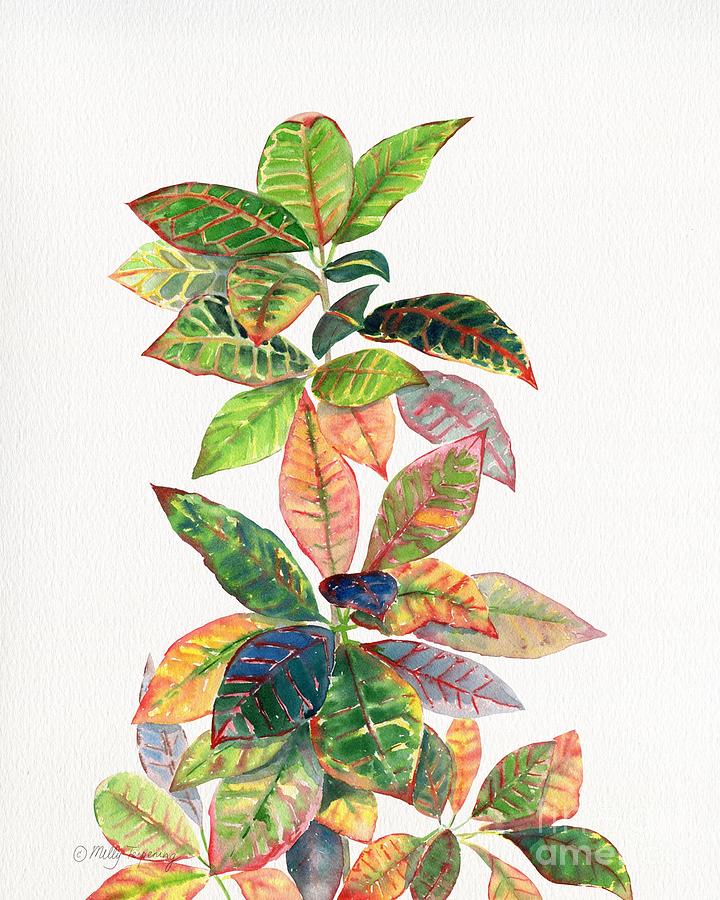This detailed watercolor painting by artist Molly Turpering, prominently features a vivid and colorful croton houseplant. Set against a white textured background, the painting displays the plant's wide, veined leaves in a mesmerizing array of colors. At the top, three distinct leaves catch the viewer’s eye: the central leaf is a blend of green with yellow accents, flanked by two others tinged with red and yellow hues. As you move your gaze downward, the leaves showcase a breathtaking palette, including a standout leaf in the center that is completely pink and yellow. 

Further down, some leaves exhibit hints of blue, darker greens, and various other shades. Towards the bottom of the painting, two flowery clusters of leaves form circular shapes, adding to the complexity and beauty of the composition. There are also some grayish-blue leaves with red veins, and dark green and purple leaves adding depth to the plant. The organized yet natural distribution of the leaves gives the painting a somewhat triangular shape as it narrows towards the top. 

In the bottom left corner, the artist’s watermark "MOLLY TURPERING" in cursive adds authenticity and personal touch, while another watermark labeled "AME" resides in the bottom right corner, both subtly blending into the serene yet vibrant composition.